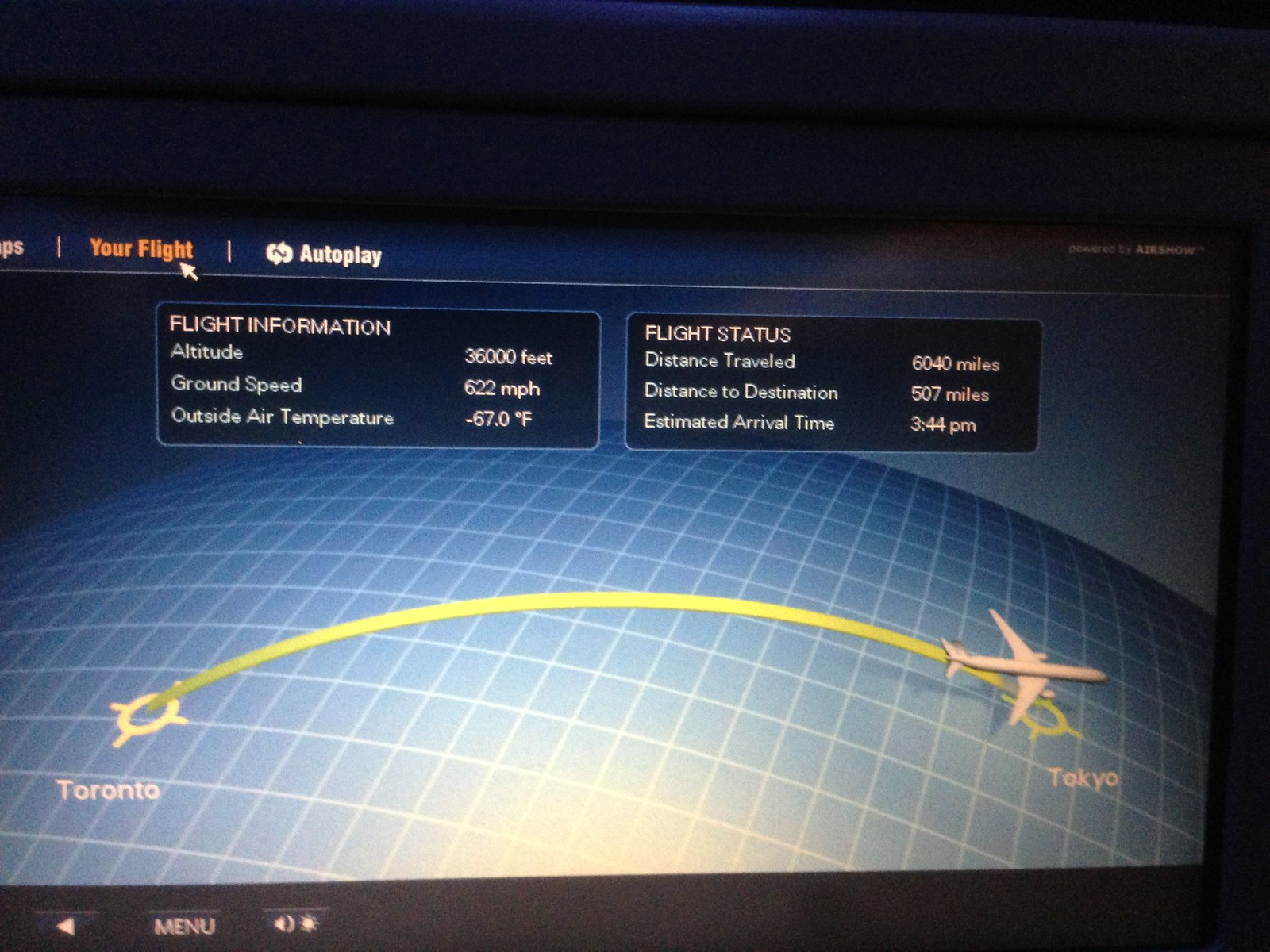The photo depicts an in-flight information display from a flight traveling from Toronto to Tokyo. Dominating the screen are two primary boxes of information: "Flight Information" and "Flight Status." The "Flight Information" box lists an altitude of 36,000 feet, a ground speed of 622 miles per hour, and an outside air temperature of -67°F. The "Flight Status" box indicates the flight has traveled 6,040 miles, with 507 miles remaining to its destination, and an estimated arrival time of 3:44 PM. The screen also features a globe image with a flight path marked from Toronto to Tokyo. The display's aesthetics are predominantly blue and white, with some text highlighted in orange. Additional visual elements include a thin bluish light at the top, suggesting the edge of a seat or a similar structure, and some partial text cut off on the left side. This older display, likely from around 2010 to 2015, shows the flight nearing its conclusion but still maintaining cruising altitude.